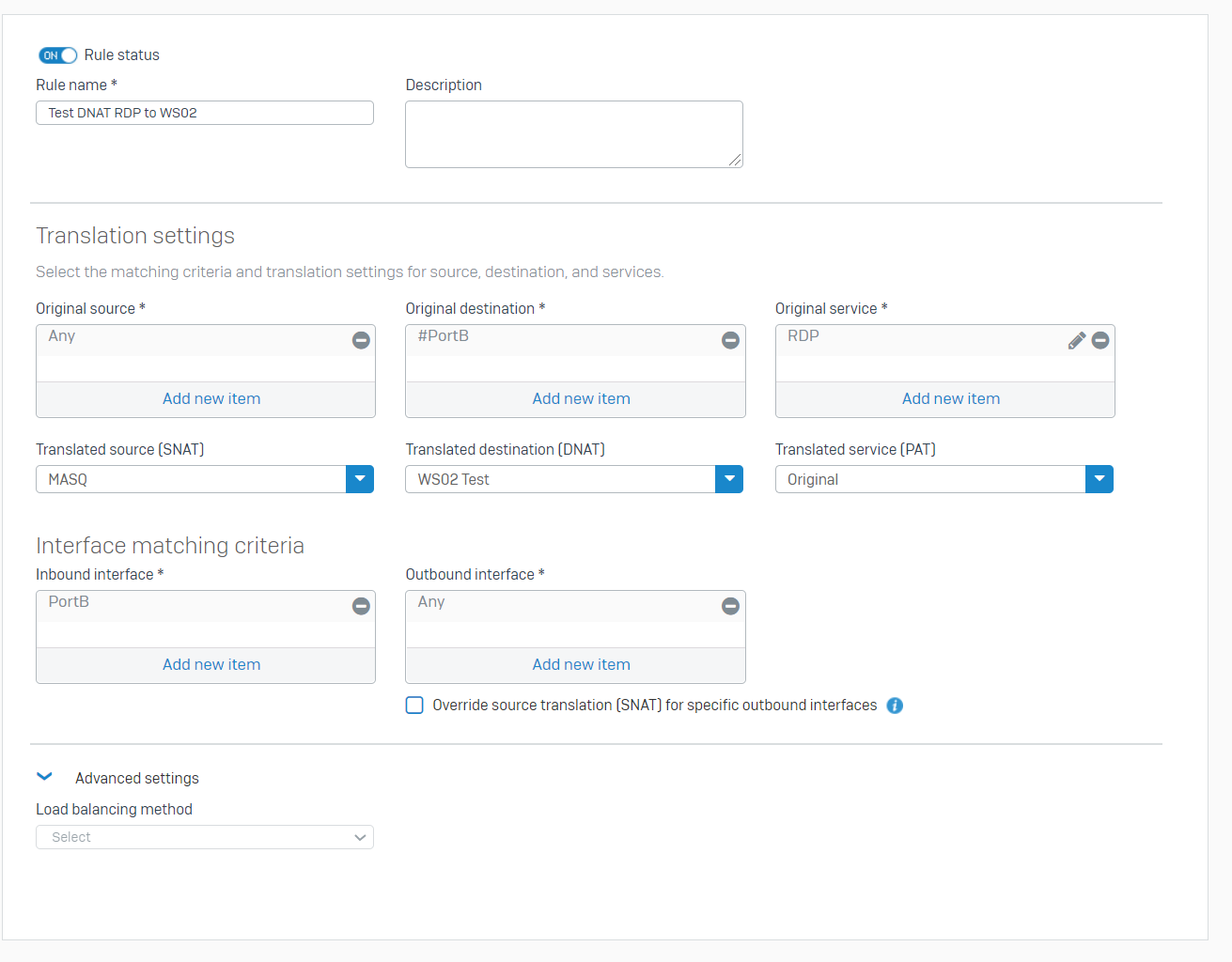The screenshot is predominantly characterized by a clean, white background encompassed by a thin gray border. This border is further accentuated by a subtle gray shadow-like effect on its top, right, and bottom sides. Positioned in the upper left-hand corner is an On/Off toggle button, currently set to "On" and highlighted by a blue background adjacent to the label "Rule Status." 

Below this label are two horizontal data entry fields. The first field, labeled "Rule Name," contains the text "test dnat rdp to ws02." The second field, labeled "Description," is positioned immediately to the right of the first. 

Central to the page is the section titled "Translation Settings," which instructs the user to "Select the matching criteria and translation settings for source, destination, and services." Here, three horizontally aligned data entry boxes labeled "Original Source," "Original Destination," and "Original Service" are clearly presented.

Directly beneath these data entry boxes are three corresponding drop-down menus labeled "Translated Source (SNAT)," "Translated Destination (DNAT)," and "Translated Service (PAT)," arranged in the same horizontal fashion.

Continuing down the page, another section labeled "Interface Matching Criteria" is visible, featuring two more data entry fields. The left field is designated for the "Inbound Interface," while the right field is for the "Outbound Interface." Underneath the "Outbound Interface" field, a checkbox option is available for "Override Source Translation (SNAT) for Specific Outbound Interfaces."

Finally, at the bottom-left corner of the page, there's an option provided for accessing "Advanced Settings."